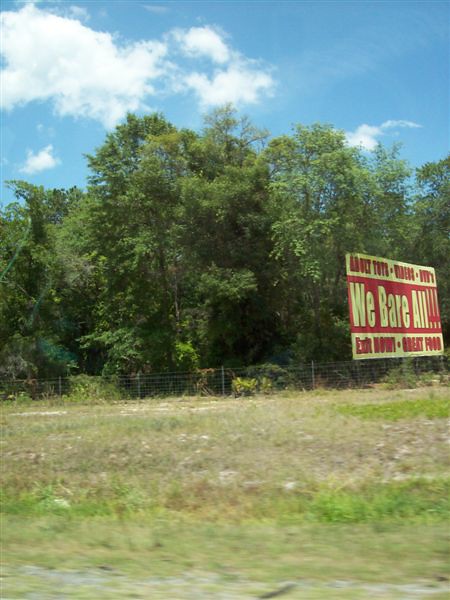The image captures a sprawling grassy field, where rocks scatter across the foreground leading into sparser brown grass interspersed with small patches of green. The field eventually transitions into thicker grass as it moves towards the chain-linked fence at the far end. Behind the fence lies a bushy and wooded area, brimming with lush green trees of varying shades.

Prominently displayed to the right of the field, beyond the fence, is a billboard. The billboard reads, "Adult Toys, We Bare All!!!, Exit Now, Great Food," with "We Bare All!!!" in white letters against a red background. The remaining text is in red letters on white backgrounds. This signage, though slightly blurry, is vibrant against the backdrop of the thick foliage.

Above it all, the scene is capped by a beautiful blue sky speckled with white, wispy clouds, lending a serene atmosphere to the initially calm but somewhat neglected landscape. The overall impression is one of a rural roadside setting, transitioning from open, untended land to a wooded area, marked by the striking presence of the billboard that advertises with bold messages and vivid colors.